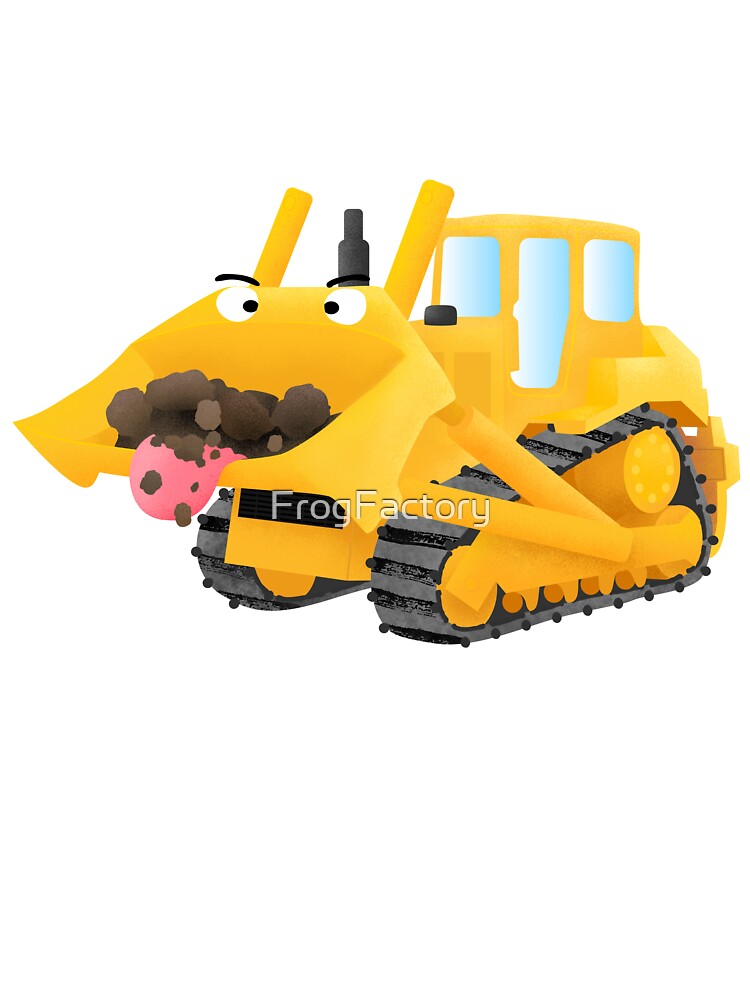This image is a detailed cartoonish illustration of a yellow bulldozer, titled “Frog Factory” as indicated by a gray watermark across the middle. The bulldozer features a cab with three windows, one serving as a door. The vehicle is equipped with large black and gray tracks and a prominent hydraulic lift system to manage the front scoop. The scoop itself, resembling a face, is filled with clumps of dirt and adorned with two expressive eyes, complete with menacing black eyebrows, and a human-like tongue sticking out, as if the bulldozer is playfully licking up the dirt. Above the scoop, there is a smokestack. The background of the image is entirely white, keeping the focus solely on the vividly detailed and anthropomorphized construction vehicle. This visually engaging and imaginative bulldozer illustration seems designed to appeal to children, possibly as a playful promotional image for Frog Factory.